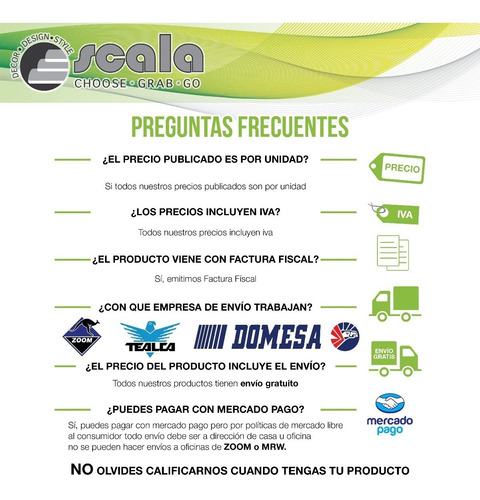The image depicts a well-organized flyer written entirely in Spanish, likely functioning as an advertisement. Prominently featuring a dark-to-light gradient of greens, blues, gray, and black, the flyer includes diverse visuals and several scattered text elements. The top left section showcases a company logo, characterized by a green-yellowish and white swirl encircling a circular icon. Adjacent to this logo, the word "scala" is printed, followed by a slogan "choose, grab, go."

The layout also incorporates various images: envelopes symbolizing communication or mail services, a truck likely indicating delivery or logistics, and an illustration of hands shaking that could imply partnerships or agreements. Text sections include notable phrases such as "preguntes frecuentes" in bold green print. Despite the scattered arrangement of the elements, the flyer maintains an overall organized structure, visually enhanced by a cohesive color palette and well-placed design elements.